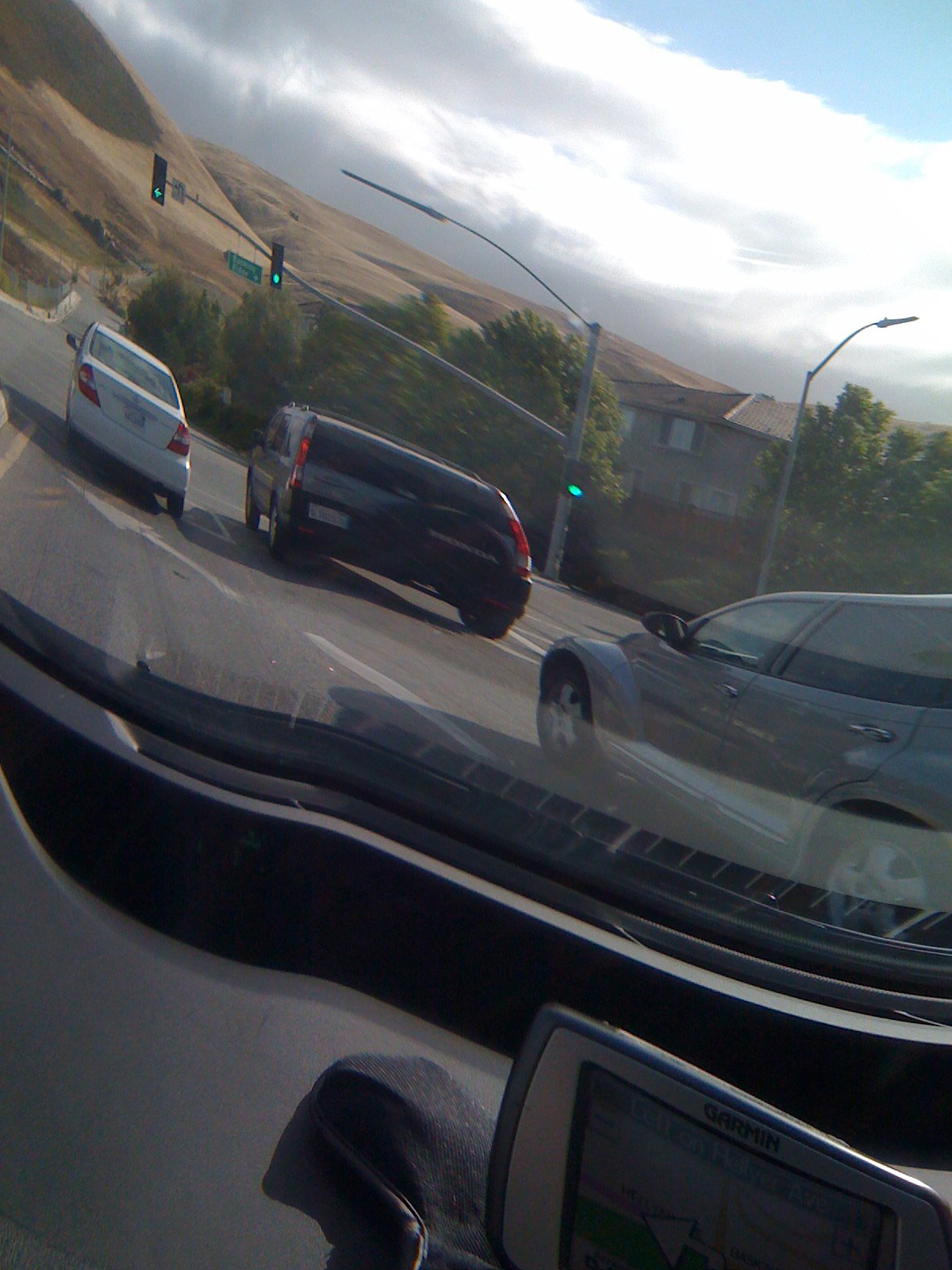This image, likely AI-generated due to its wavy and diagonal distortion, captures a daytime street scene through the windshield of a vehicle. The dashboard, dark grey with a black trim around the windshield, prominently features a silver GPS device with a blue housing, faintly displaying the brand name "Garmin." The vehicle is stopped at an intersection, evident from the visible dashboard screen and part of the rearview mirror. 

In the foreground, three cars are noticeable: a gray van to the right, a silver SUV stopped at the light, and a white sedan directly in front. The traffic lights are green, with one displaying a green arrow and another a green dot, alongside a small green crosswalk light. A green street sign with white lettering hangs from the traffic light but remains unreadable. 

The background features a mix of urban and natural elements, with light brown, golden brown, and dark brown hills stretching out beneath an overcast sky dotted with fluffy white clouds and patches of blue. The right side of the scene presents grey and white buildings, one with a dark brown roof and fencing, nestled among dark green trees. Road markings, including white arrows, stand out against the light grey asphalt. Additionally, there are street lamps and a secondary light pole, indicating nighttime street illumination. A fence lines the left side of the road, framed by patches of light green and grey grass.